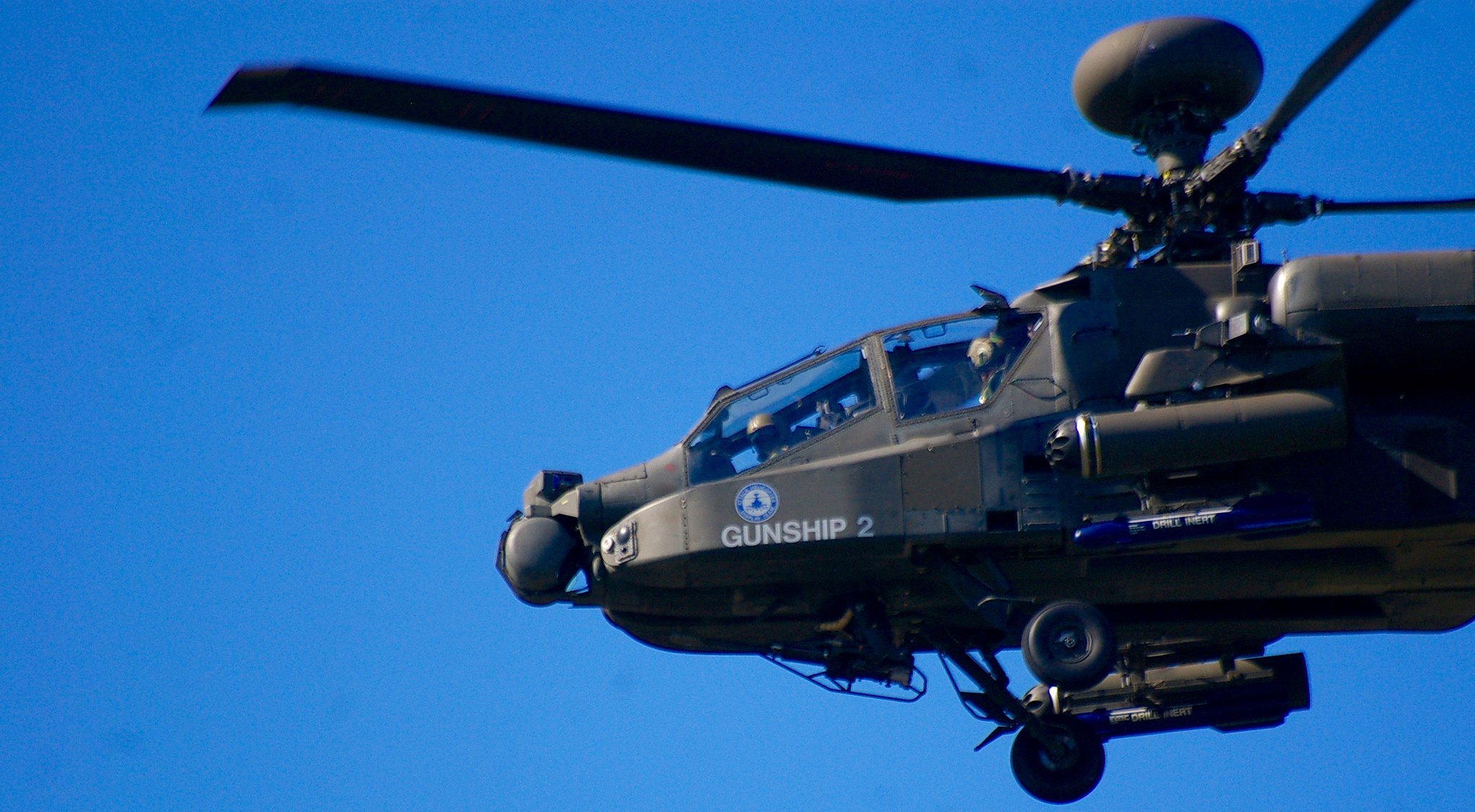This photograph captures a sleek, modern attack helicopter in mid-flight against a perfect, cloudless blue sky. The helicopter, predominantly black in color, prominently displays the text "Gunship 2" in white stencil lettering on its front. Above the text, there is a blue and white emblem, possibly military in nature. The aircraft's main rotor blades are clearly visible and appear to be in motion. The pilot, and potentially a co-pilot, can be seen through the front and side windows of the cockpit. The helicopter's landing gear is clearly off the ground, emphasizing that it is airborne. Additional details include various cylindrical components and a payload located under the helicopter, suggesting its armed forces designation. Overall, the image showcases the helicopter's powerful and modern design.